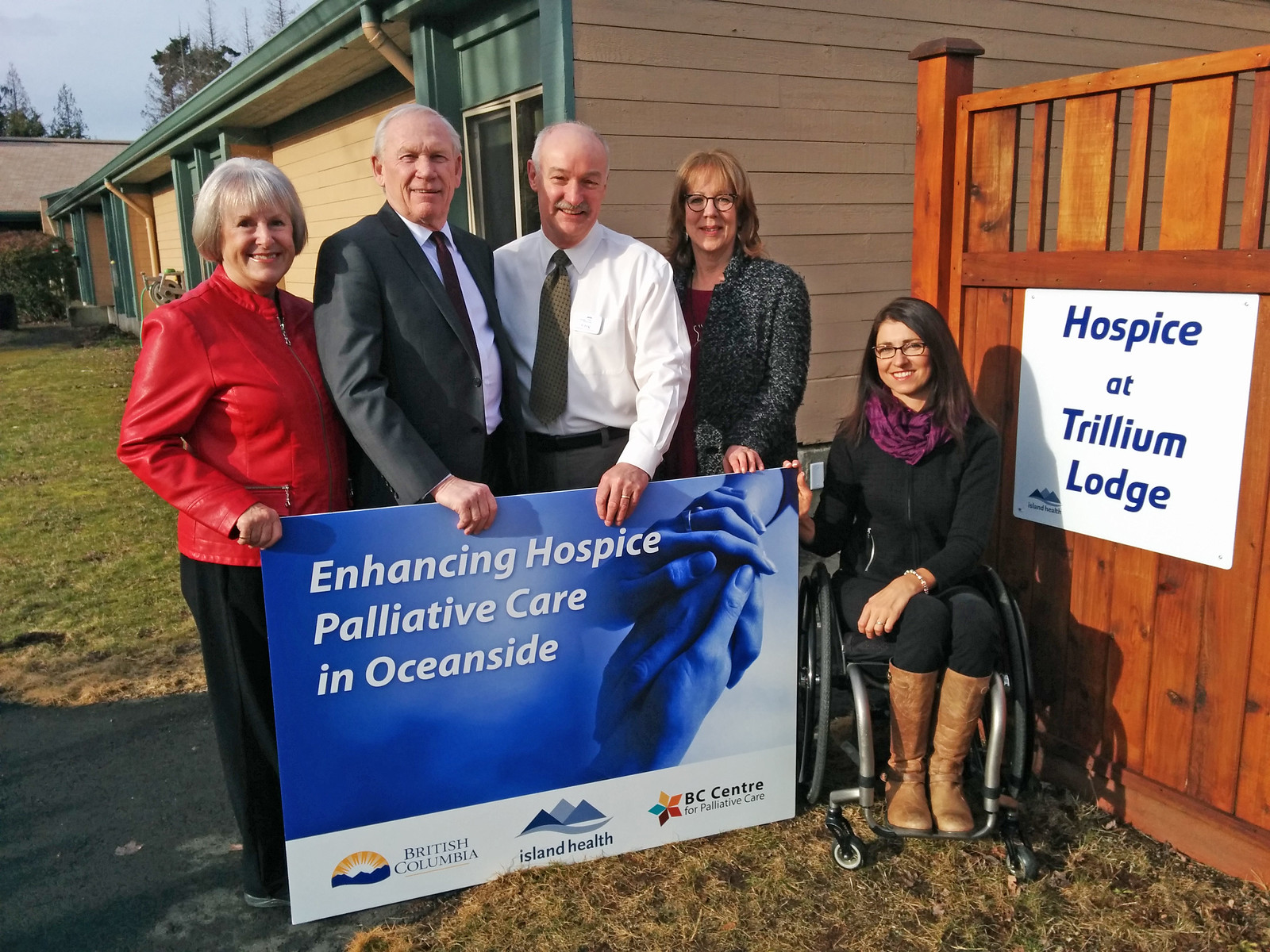Five individuals are gathered outside on a pleasant day in British Columbia, posing in front of a building associated with a hospice home, as indicated by the brown fence nearby labeled "Hospice at Trillium Lodge." They are holding a large sign inscribed with "Enhancing Hospice Palliative Care in Oceanside," featuring an image of hands holding each other and logos for British Columbia Island Health and the BC Centre for Palliative Care.

The group consists of four older individuals standing behind the sign and a younger woman in a wheelchair to the right. The first person on the left is a woman in her 60s, recognizable by her red leather coat and black pants, with short gray hair. Next to her stands an elderly man in a dark gray suit, complete with a tie. Adjacent to him is another older man dressed in a white dress shirt with a green tie and short gray hair. Then, a woman with medium-length brown hair and glasses wears a heathered gray jacket. Finally, on the far right, is a younger woman in a black jacket, brown boots, and a purple scarf, seated in a wheelchair.